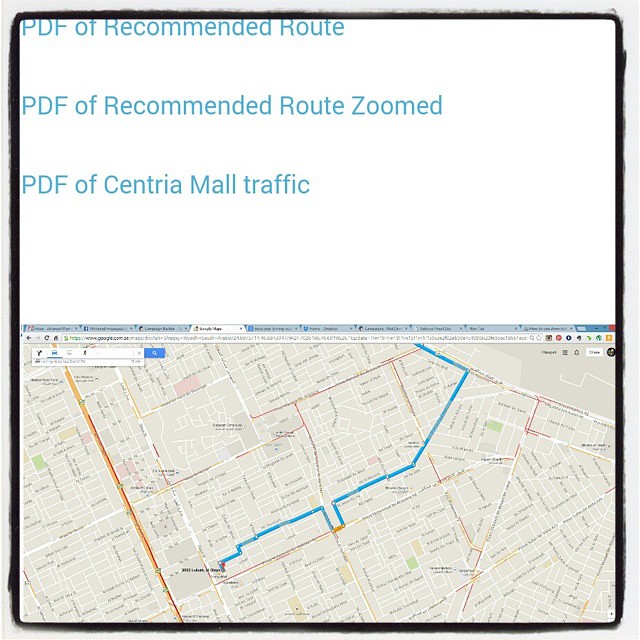This image is a detailed screenshot of a PDF file displaying directions on a Google Map. The bottom half of the image features a map with a prominent blue route line diagonally traversing the middle, highlighting the path to a specific destination. The map itself is a gray background with streets in white and a highway marked in orange and red. At the top half of the image, the text prominently reads: "PDF of Recommended Route," "PDF of Recommended Route Zoomed," and "PDF of Sentria Mall Traffic." Additionally, there are multiple tabs open, including Facebook, visible at the top of the screen. The image captures the detailed layout of the map, showcasing streets, interstate routes, and the toolbar, all over a light beige background.